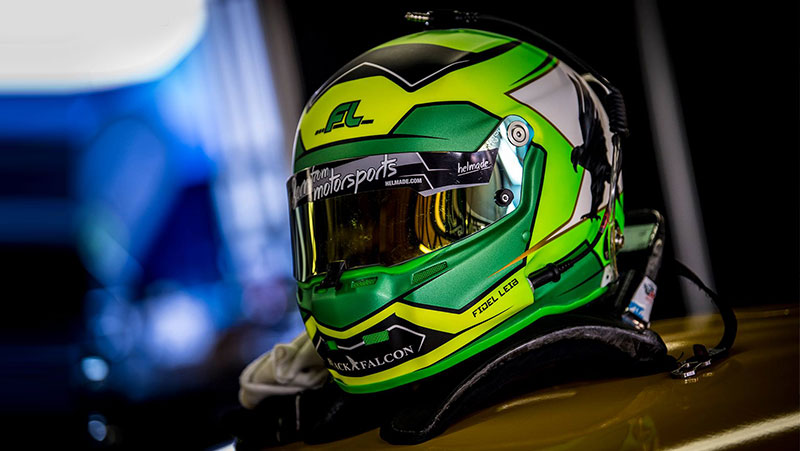This horizontal photograph captures a racing helmet as its central focus. The background is blurred, displaying a gradient of colors: dark blues and whites towards the left, transitioning to black with a beam of white light on the right, and a gold metallic hue in the bottom right corner, indicative of a car. 

The helmet, prominently positioned, is adorned with a vibrant combination of colors. Primarily showcasing shades of bright lime green and dark green, it features black and white sections as well. The top of the helmet bears the initials "FL" in green letters, outlined in black, aligned above an obscured word followed by "Motorsports." On the visor, "Motorsports" is clearly inscribed, and near the chin area, the words "Black Falcon" and "Fidel Leia" (spelled L-E-I-A) are visible.

The helmet's design includes a dark green area outlined in black near the visor, with the rest of the helmet covered in a striking yellow-green hue, reminiscent of Mountain Dew. The helmet extends down past the chin, merging into a black cushion that appears to be attached to a gold-topped car.